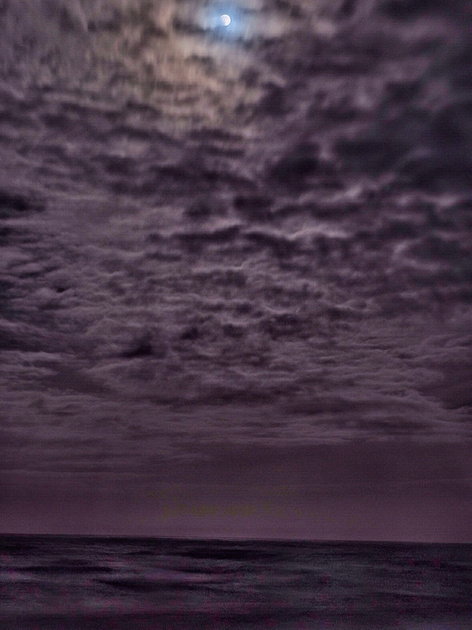The image captures a somewhat blurry nighttime seascape bathed in various shades of purplish-gray. At the top middle of the photo, a small, bright moon peeks out from behind thick cloud cover, which is tinged with bluish hues and lighter whitish-gray areas. The horizon, slightly slanted, separates the dark, slightly wavy sea from the sky. The water at the bottom of the image displays a grayish-blue tone, occupying only a small portion of the overall scene. Above the horizon stretches a vast expanse of clouds, gradually becoming closer and more detailed as they approach the top of the image. The entire photograph is tinged with a granular effect, emphasizing different gradations of purple from the sea to the sky, making the moon's luminous presence all the more striking against the dark, cloudy backdrop.